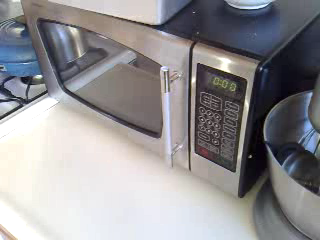This is a close-up color photograph of a digitally controlled microwave oven situated in a kitchen. The microwave has a sleek silver exterior with a glass front and a silver door handle, set within a predominantly black control panel featuring white-outlined buttons. The digital display shows a time of 00:00 in a greenish-yellow hue. The microwave sits on a pristine white countertop, with various unspecified items stored on top of it. To the right of the microwave stands a metal mixing bowl, likely part of a small mixer. In the background, just to the left of the microwave, is a gas stove top with a blue pot positioned on one of the burners. The scene captures a glimpse of everyday kitchen appliances in a well-organized space.